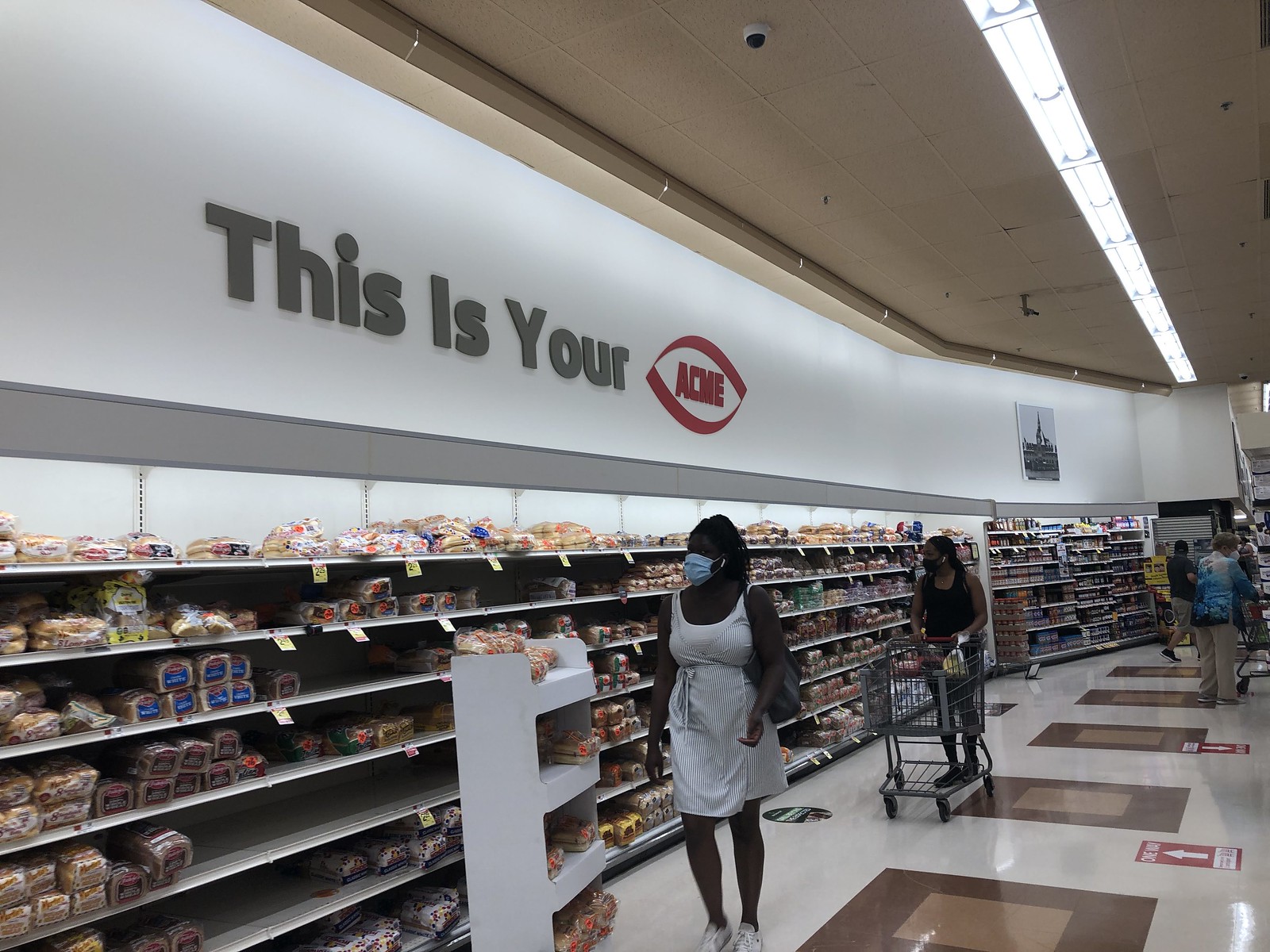The image captures an interior view of an Acme supermarket during the Covid era, evident from the face masks worn by the individuals. The setting is a spacious bread aisle located along the perimeter of the store, which features an extensive shelving system stacked with various types of bread and bagels. Overhead, the sign reads "This is Your Acme" in gray and red letters, enclosed in a red lemon-shaped outline. The ceiling is adorned with bright lighting fixtures that span the aisle's length and is equipped with a few security cameras.

In the foreground, a dark-skinned black woman is wearing a white dress with blue print, a light blue mask, and white sneakers. She carries a black handbag and seems to be inspecting the bread. Standing about six feet behind her is another black woman with lighter skin, dressed in a black cami, black shorts, and black sneakers. She has ear pods in, a black mask on, and is pushing a grocery cart containing bananas and other produce. Further behind, an elderly man in a tropical-colored shirt and khaki pants, also pushing a cart, is turned away from the bread aisle. Lastly, a younger man in a black t-shirt and brown cargo shorts is seen in the distance, facing away from the camera as if looking towards another section of the store.

The floor features a decorative pattern of brown squares bordered by darker brown squares, adding a subtle aesthetic to the supermarket's clean and organized appearance.